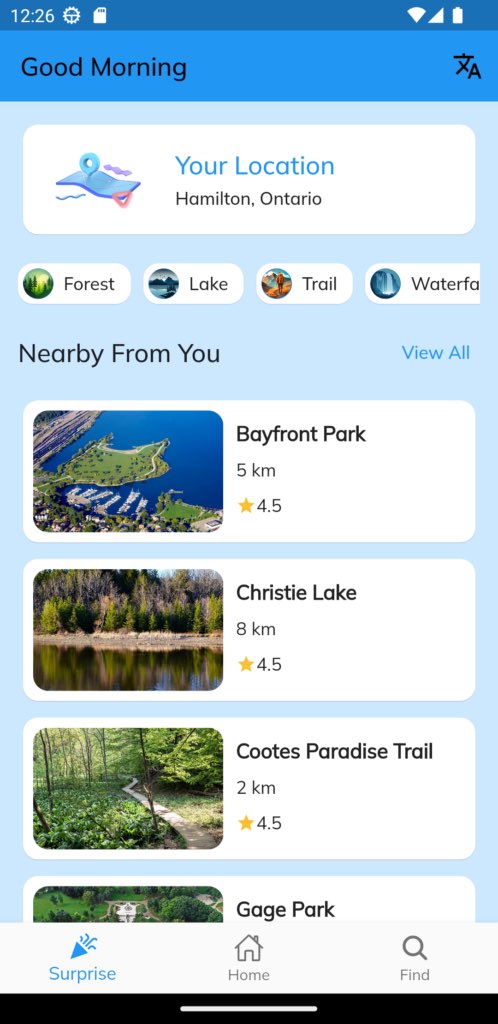"This is a screenshot of the front page of an outdoor app. At the top center of the screen, there is a horizontal row of categories labeled 'Forest,' 'Lake,' 'Trail,' and 'Waterfall.' Directly above this row, there is a white search box with the placeholder text 'Your location,' and slightly below it, in small black letters, it reads 'Hamilton, Ontario.'

In the lower center of the screen, to the left, the text 'Nearby from you' is displayed, while to the right, in small blue letters, it reads 'View All.' Below this section, there is a vertical list of different outdoor areas, each featuring detailed information and small thumbnails.

The first listing is contained within a white rectangular box displaying an aerial image of a park. To the right of the image, the text reads 'Bayfront Park,' with a distance of '5KM' and a star rating of '4.5 stars.'

The second listing follows a similar format, with another white box showcasing an image of a lake. To its right, the text indicates 'Christie Lake,' '8KM,' and '4.5 stars.'

The third listing displays a trail through a park, with the accompanying label 'Cootes Paradise Trail,' '2KM,' and '4.5 stars.'

At the very bottom of the list, there is a partially visible white box with the top portion of an image and the text 'Gage Park'; the rest of this entry is cut off.

At the very bottom of the screenshot, there is a horizontal row of navigation icons. The first icon on the left, labeled 'Surprise,' is highlighted in blue. The center icon reads 'Home,' and the icon on the far right is labeled 'Find.'"